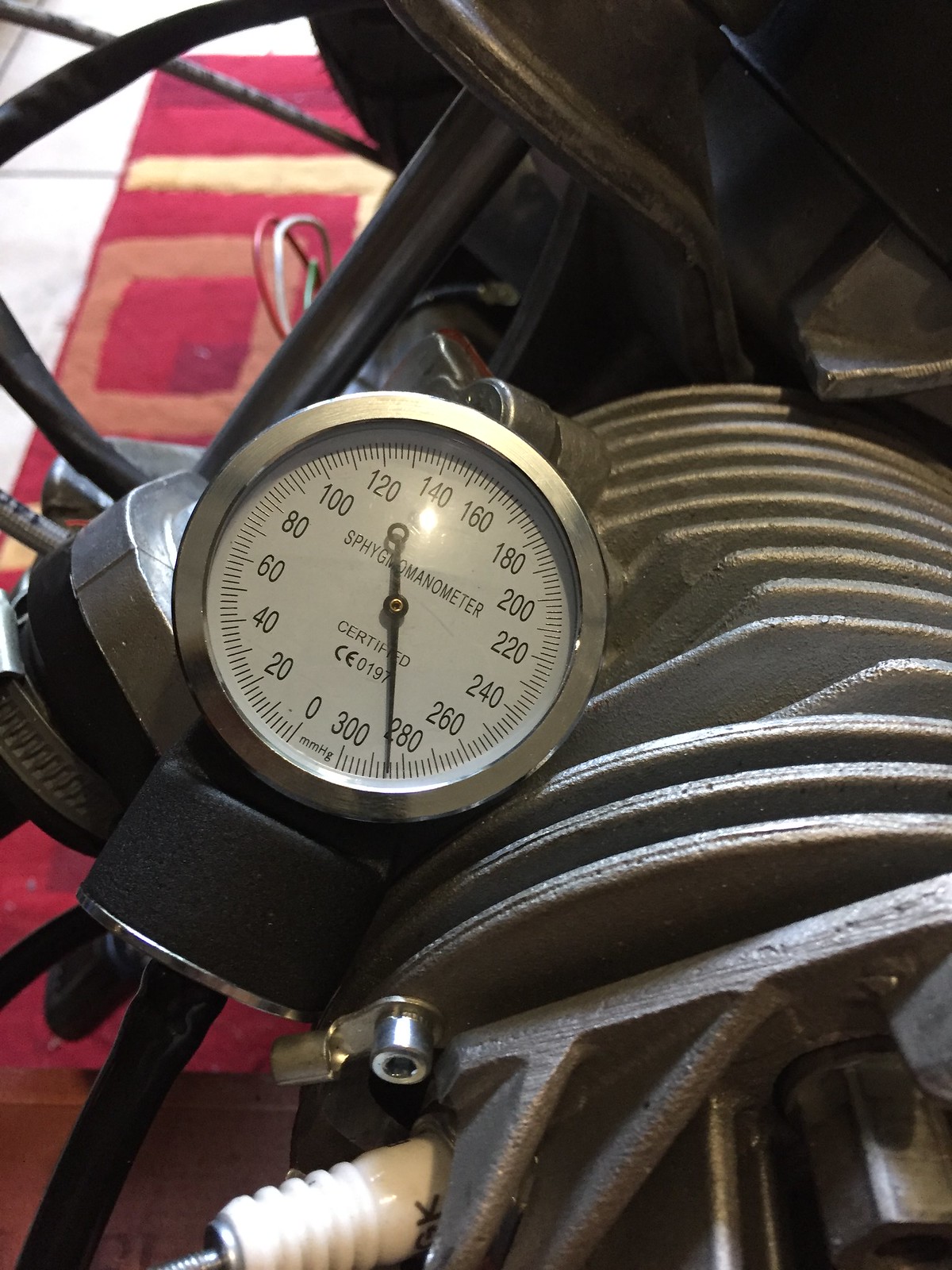The image prominently features a sphygmomanometer gauge situated centrally on what appears to be an engine. The sphygmomanometer, clearly labeled and marked from 0 to 300 in increments of 20, dominates the visual field, particularly its certified markings in the center. To the right of the gauge, there's a conspicuous engine block made of metal, characterized by distinct ribbing and circular metallic appendages. A white piston, situated at the bottom of the image, fits snugly into the engine block, which itself appears robust and mechanically intricate.

The background includes a red carpet, adding a stark contrast to the metallic elements, and possibly more metallic components that resemble pistons at the top of the image. There's also a bolt near a white plug at the bottom, and various metal brackets on the left side. The scene is completed with the presence of white tile on the left portion of the image, contributing to an industrial, mechanical environment.

Overall, the image is a detailed snapshot of a mechanical setup, focusing intensely on the gauge and its surrounding engine components.